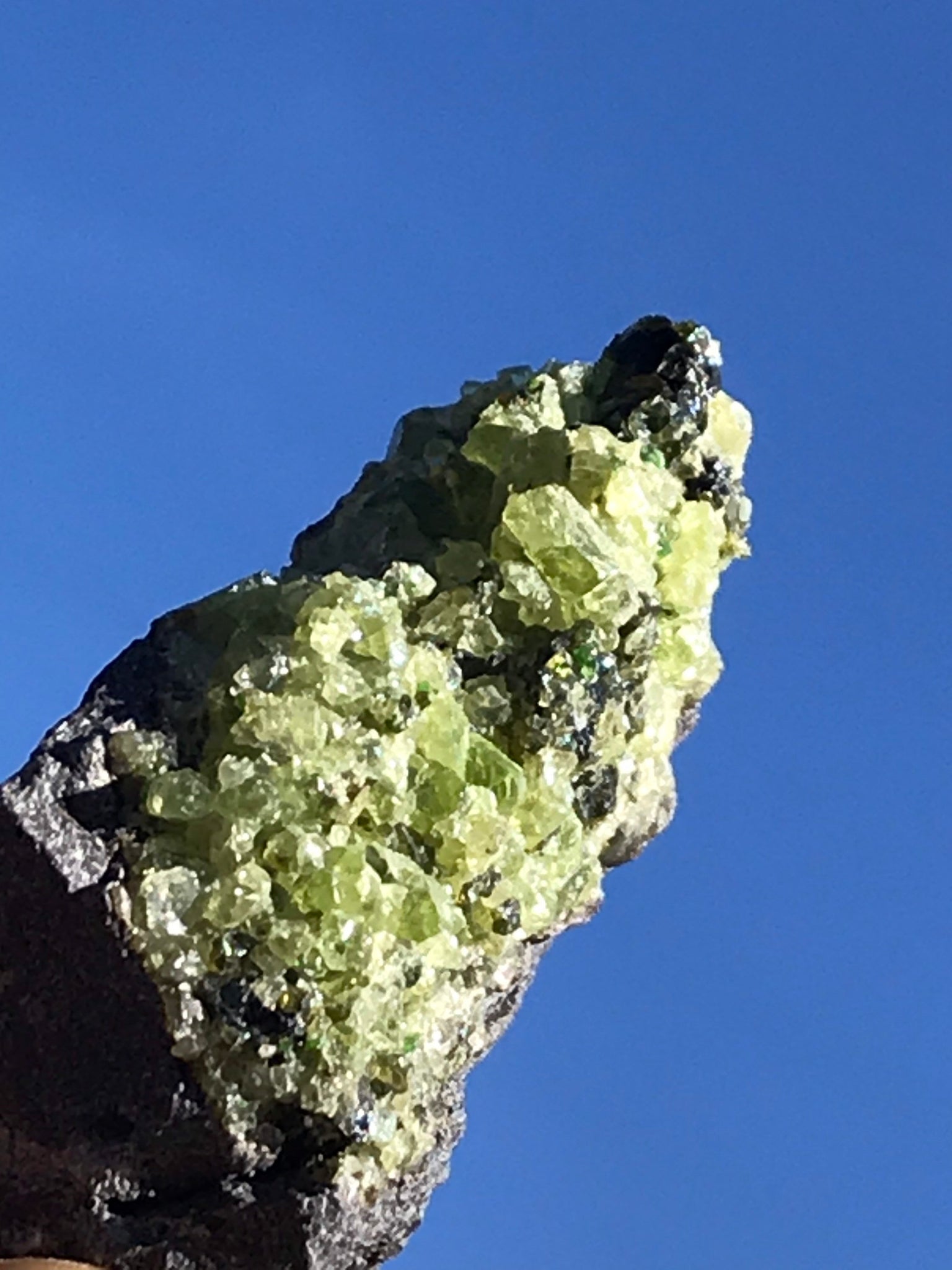This is a detailed photograph of a large, brownish-gray rock with striking crystal formations. Emerging from the lower left corner of the image and extending towards the center, the rock is adorned with clusters of vibrant yellow and emerald-green crystals. These crystals appear jagged, with their edges transitioning from a darker green to a frosted white, hinting at their layered growth. The background is a solid, pristine blue sky, giving an impression of a studio setting but likely captured outdoors. The photograph is taken in a portrait orientation, devoid of any human presence or other contextual details, focusing solely on the rock and its mineral adornments.